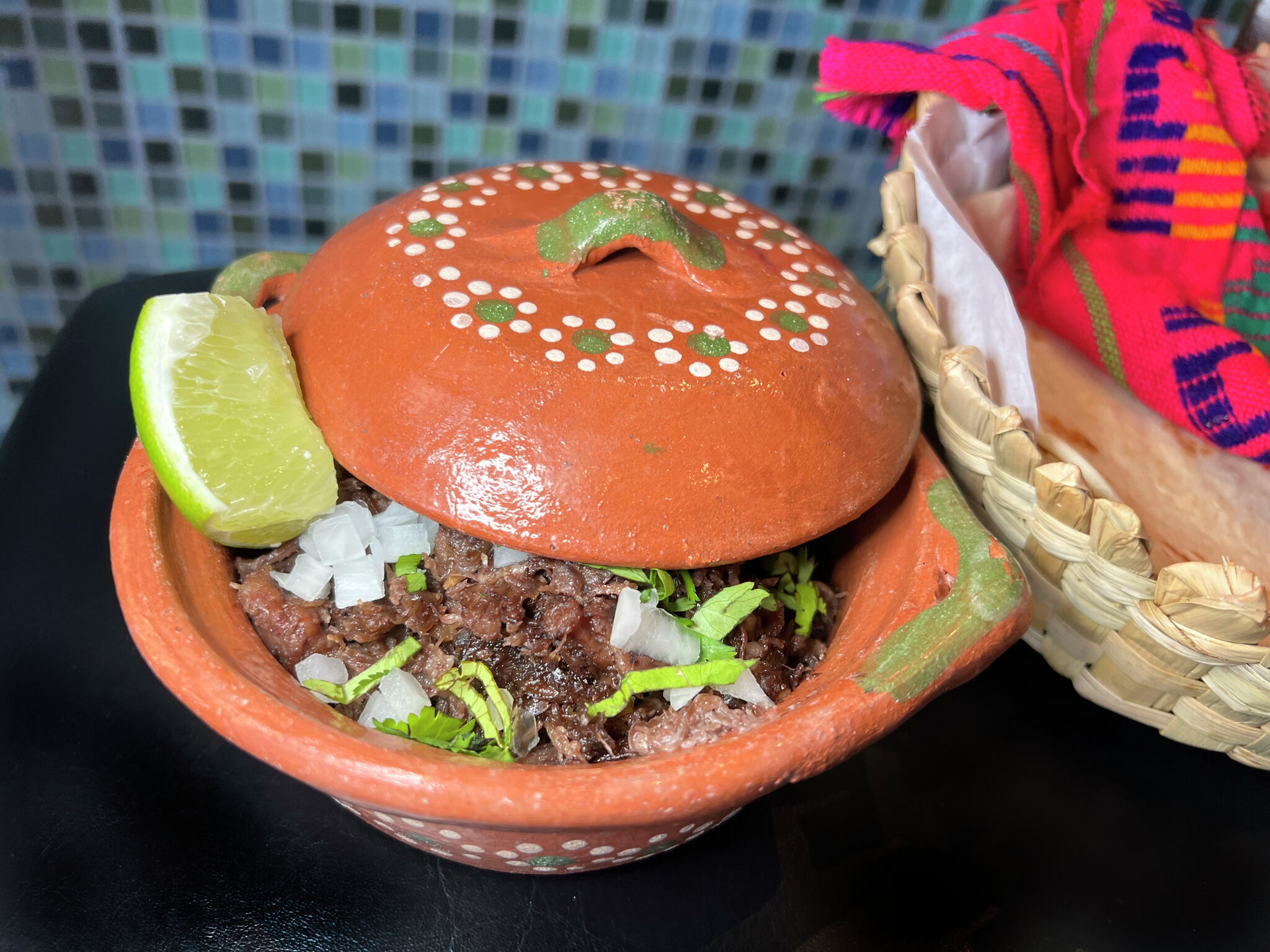This detailed close-up image depicts a vibrant culinary scene centered around a terracotta pot filled with a savory fajita mixture, comprising tender meat, chopped onions, fresh cilantro, and a tantalizing slice of lime. The pot is adorned with a charming white dot flower pattern encircling a green center, a motif that extends to its rounded, green-handled lid, which is tilted to reveal the delicious contents within. Accompanying this centerpiece is a wicker basket lined with a striking pink towel, slightly pulled back to display a stack of warm tortillas. Both the pot and the basket rest on a sleek black table, set against a backdrop of colorful mosaic tiles in shades of blue, green, and yellow, enhancing the vibrant and inviting atmosphere of the scene.